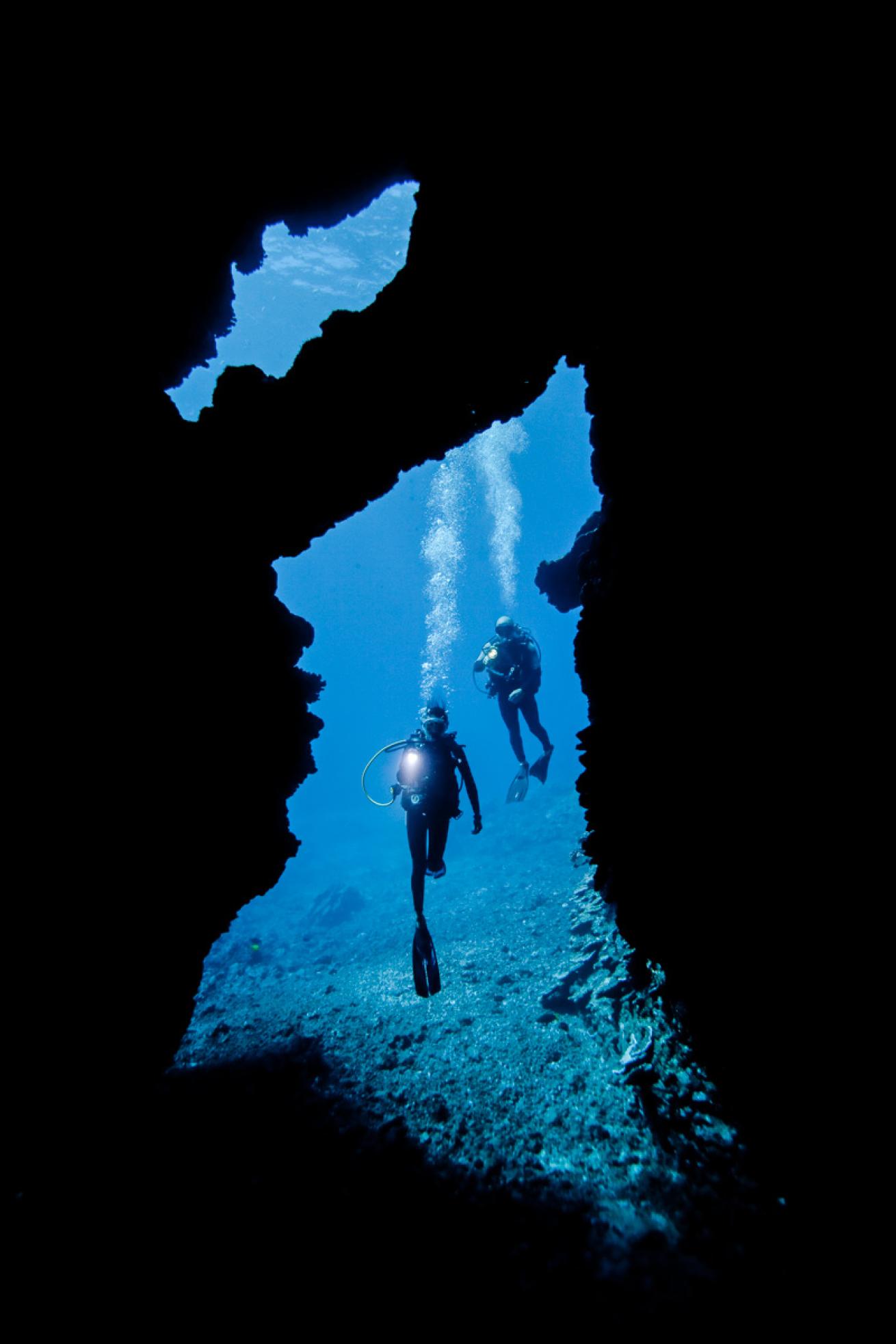This vibrant color photograph captures an underwater scene characterized by a stark black background and the brilliant blue of the ocean water. At the center of the image, two scuba divers equipped with full scuba gear, including fins, masks, and large oxygen tanks with tubing, are seen floating and making kicking motions. The diver on the right is positioned slightly higher than the one on the left. Both divers are forward-facing and peering into an underwater cave, with their flashlights illuminating the scene. Air bubbles rise from their heads, accentuating the clear, beautiful blue water around them. This appears to be a cave dive, as the photograph offers a view from within the dark, rocky entrance of the cave, where both divers are approaching. The divers are surrounded by dark rock formations and some corals at the bottom, adding depth to the underwater landscape. The scene is serene and mysterious, highlighting both the exploration and beauty of the ocean depths.